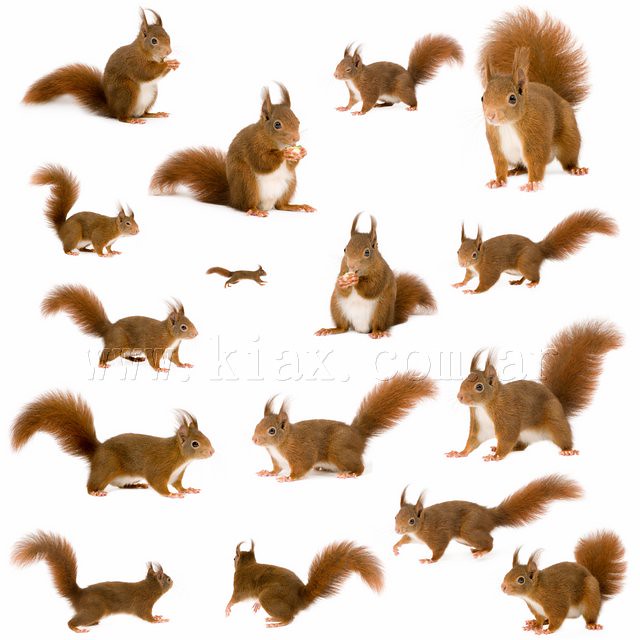This detailed image features 16 chestnut-brown squirrels arranged in rows of four against a plain white background. Each squirrel is depicted in various poses, highlighting their short, straight fur on the body and large, bushy tails. Some squirrels can be seen sitting on their haunches, nibbling on what appears to be nuts, while others are on all fours, alert and scanning their surroundings. Their distinguishing features include large, beady black eyes surrounded by a delicate white line and distinctive ears with a slight point and curvature, resembling an aerodynamic design. The squirrels exhibit a range of orientations, with some looking directly at the camera and others glancing sideways or in different directions. The image also includes a watermark at the top, reading "www.kiax.com.ar".